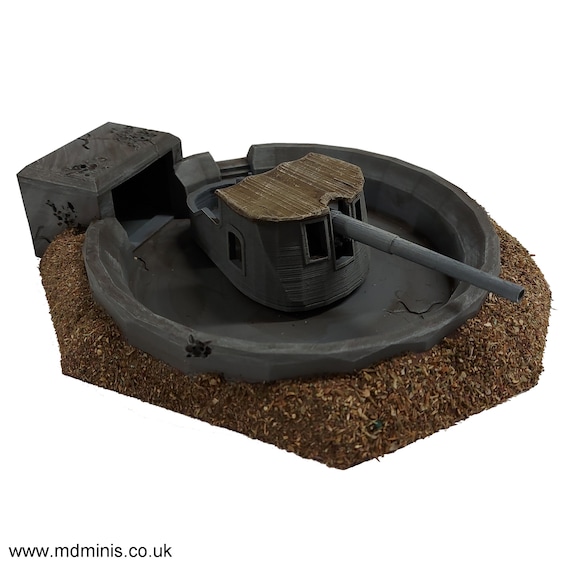The image depicts a detailed miniature model of a futuristic piece of military equipment, showcased against a white blank background. At the center of the model, there is a semi-circular shed with an elongated rifle or cannon extending toward the bottom right, resembling weaponry seen on tanks or from wartime apparatus. The shed features a flat brown thatched roof, suggesting a rustic yet tactical design. This central turret is integrated into a circular base of dark metal gray, which is mostly buried in surrounding brown dirt or mulch, enhancing the overall realism of the scene. On the left side of the model, there is a square-shaped bunker with an open front and a flat roof, adding to the fortified look. The entire model exudes a sense of historical military re-enactment or strategic equipment, meticulously crafted to display aged elements and surface cracks, possibly indicating it was carved from stone or clay and painted black. At the bottom left corner of the image, a watermark reads www.mdminis.co.uk, indicating the source or creator of the miniature. The realism and intricacy of this photographic representation capture the essence of a historical military scene or a futuristic war reenactment piece.